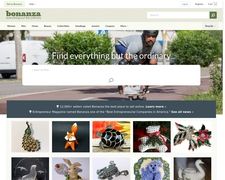This screenshot captures a section of the Bonanza website, though it is quite blurry, making identification of specific details challenging. Prominently displayed in the center is the tagline, "Find everything but the ordinary," underscored by a collage of various eclectic images. Among these images are distinct pictures such as a pineapple, a fox, a turtle, a bear, and a bird adorned with flowers, contributing to a quirky and diverse visual theme. 

In the background, a man can be seen skateboarding, adding a dynamic, adventurous element to the layout. At the top right corner of the screen, there is a search button, indicative of the website's navigational features. A faint white bar spans the top of the image, accompanied by what appears to be a secondary menu, though the details are indiscernible due to the image’s lack of clarity. The overall color scheme exudes a greenish hue, complementing the site's adventurous and naturalistic vibe.